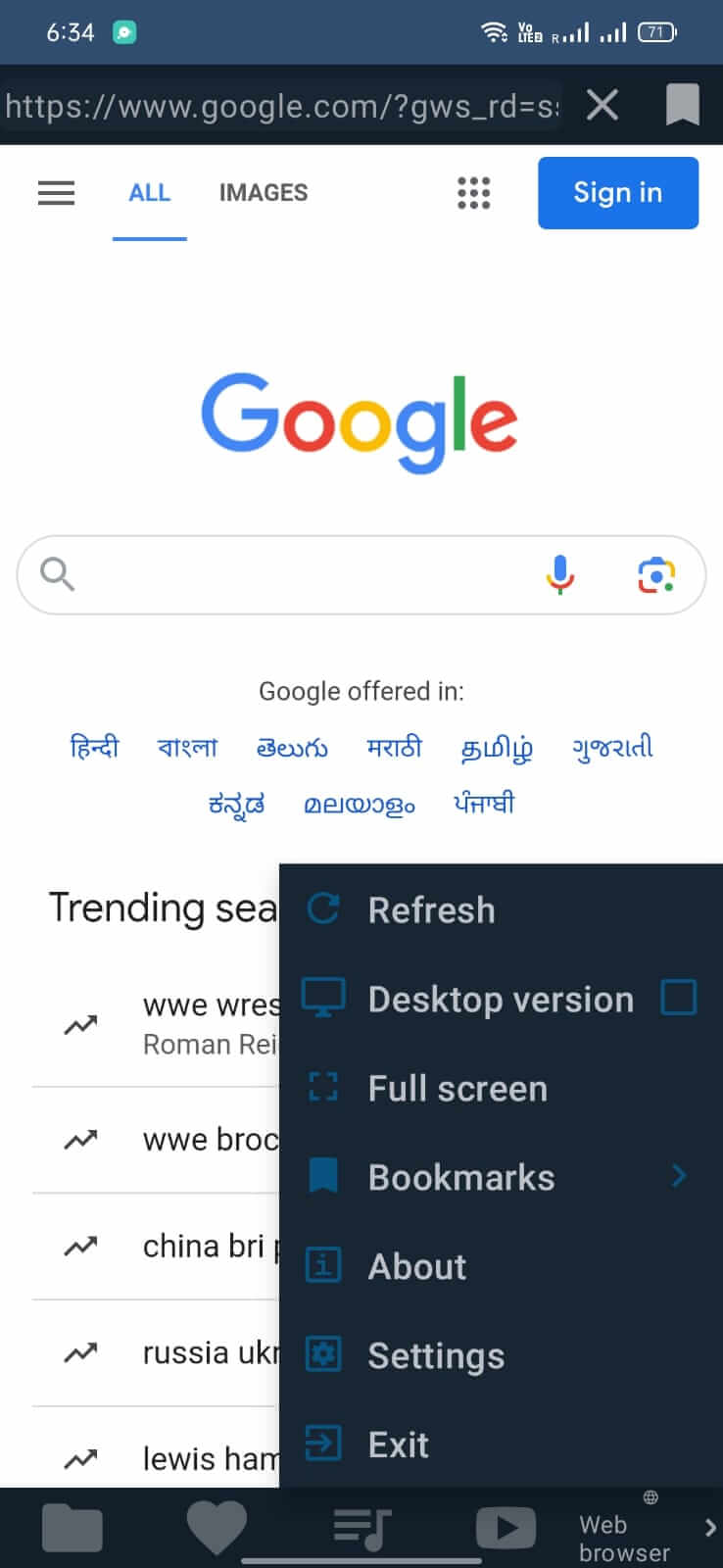Screenshot of the Google homepage on an Android device displaying the Arabic version. At the top, the iconic Google logo is prominently featured. Beneath it lies the search box, inviting users to type their queries. The current user is not signed into their Google account, as indicated on the page. A settings drawer has been opened at the bottom right, showcasing options such as "Settings," "About," "Bookmarks," "Full Screen," "Desktop Version," "Refresh," and "Exit." This settings menu partially obstructs the "Trending Searches" section, making it challenging to view the complete list of trending topics. However, some visible top searches include Roman, China, Brie, Russia, Ukraine, and Lewis Hamilton. The primary language displayed is Arabic, and the note "Google offered in" followed by multiple Arabic language options can be seen beneath the search box.